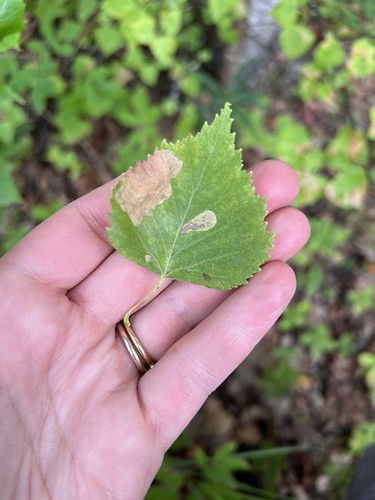A photograph captures a close-up of a person's hand emerging from the bottom left corner, extending toward the center, where it delicately holds a leaf showing signs of disease or decay. The leaf, exhibiting green and brown hues, appears to suffer from a fungal infection or plant disease. The hand, light pinkish-white, sports a double-stacked, thick gold wedding ring on the ring finger. The backdrop features a blurry blend of green foliage and dark brown leaves or soil, indicative of a forest floor. The scene is set outdoors in daylight, with the natural surroundings softly blurred to emphasize the central subjects: the hand and the leaf. The photo contains no text and presents a color palette of green, brown, beige, gold, black, and gray.